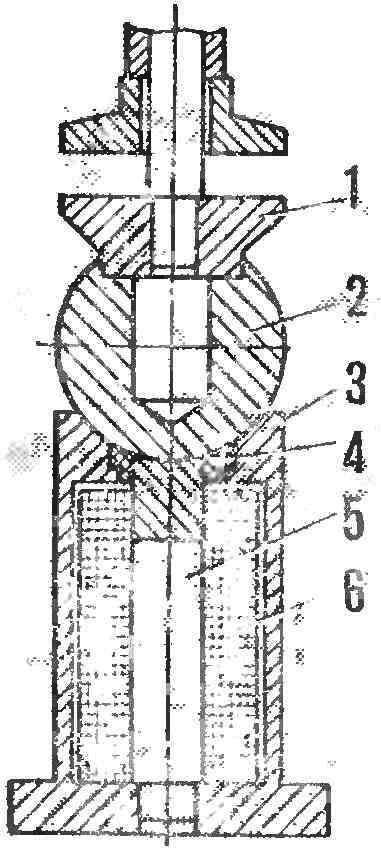The image is a detailed black and white technical drawing, likely an engineering schematic, featuring a tall vertical structure depicted in a side view. The drawing is labeled with the numbers 1 through 6, each pointing to different sections of the structure. The image is a cutaway view, revealing the interior and various components of the object. The drawing comprises several geometric shapes: a horizontal rectangle at the bottom for stability, overlaid by a vertical rectangle, a circle, and two trapezoidal shapes stacked sequentially on top. This structured depiction includes lines shading different areas, indicating variations in material or functionality. The top section appears to have an area for a bolt or screw, possibly for assembly purposes, while the bottom, wider section may serve as a stable base. The overall composition is arranged to show different parts that are presumably assembled together, illustrating an intricate piece of heavy machinery, perhaps a press, with a piston-like component at the top.